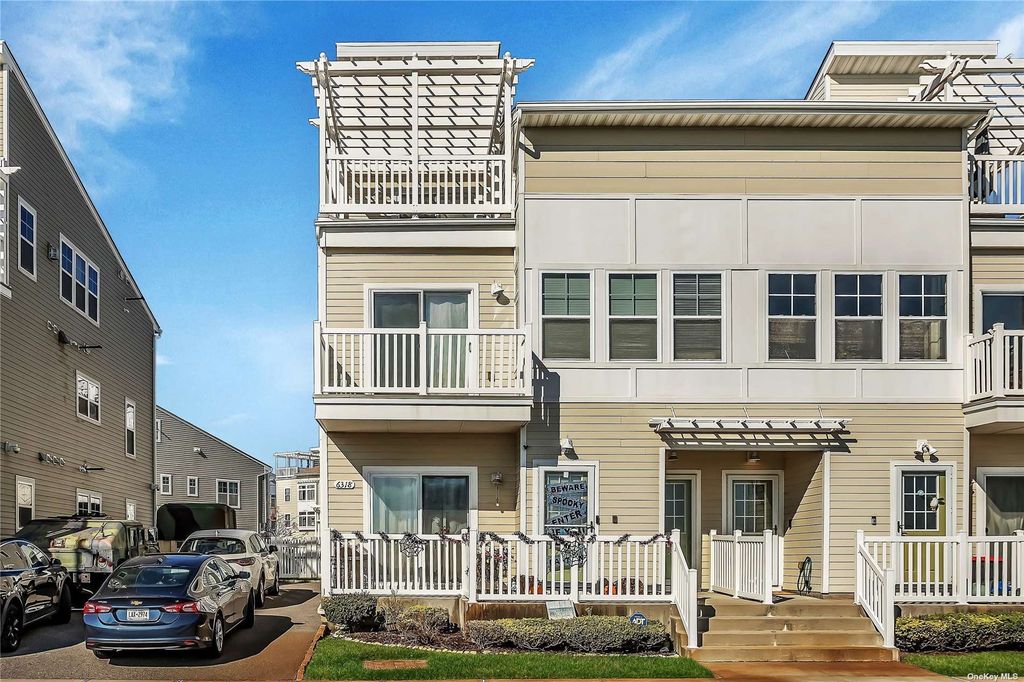The photograph captures a large, modern, beachy house that appears to be a two-story or possibly three-story structure. The house is characterized by its beige wood paneling and white accents, giving it a contemporary aesthetic. The facade features several windows, and balconies are present on each level, with some balconies protected by white railings. A distinct division can be seen between the left and right sides of the house, hinting at a possible dual-occupancy setup, potentially suggesting it could be a condo or an apartment.

The top portion of the house, featuring a small balcony with a roof, adds to its charm. The middle floor boasts six windows lined in a row, and sliding glass doors leading to decks on each floor. At the entrance, a staircase is flanked by Halloween decorations, including a prominent spider web and a "beware spooky enter" sign over one of the doors, adding a festive touch.

In front of the house, well-manicured lawns and flower beds offer a splash of greenery, complemented by additional shrubbery. Three cars—a white SUV, a blue car, and a black car—are parked next to the house. To the left, the edges of similarly styled homes are visible, painted in shades of tan and gray. The entire scene is set against a backdrop of a clear, blue sky, indicating a bright and sunny day.